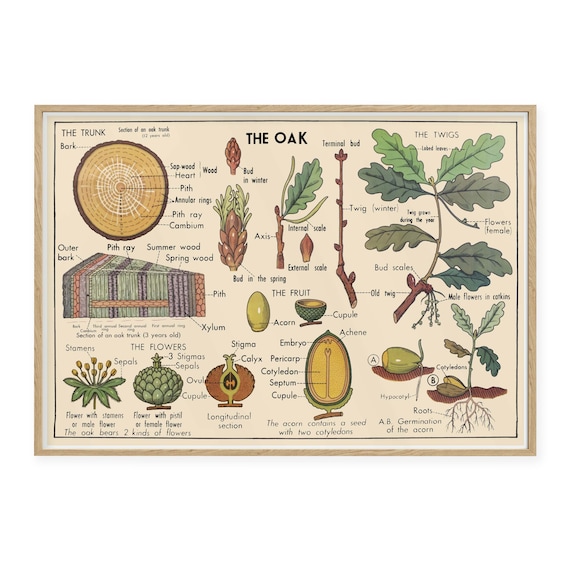The image is a detailed botanical chart of an oak tree, meticulously framed with a thin, light brown wooden border. Measuring approximately three inches wide and two inches high, it features three distinct borders: the outer wooden frame, a pinstripe white inner border, and a recessed light tan paper border with a black pinstripe. At the top of the chart, bold black letters spell out "The Oak."

The central section of the chart focuses on the anatomical components of the oak tree. In the upper left corner, there is a labeled depiction of the trunk showing a cross-section that highlights the bark, sapwood, heart, pith, annual rings, pith ray, and cambium. Below this, a pie-shaped wedge illustrates the outer bark, summerwood, springwood, pith, xylem, and other minute structures. The lower left corner of the chart features the oak's flowers, including stamens or male flowers on the left and various labeled parts like stigmas and sepals on the right.

The bottom section explains that the acorn contains a seed with two cotyledons, detailing components such as the etchian embryo, pericarp, cotyledon, septum, and capule. Also in the lower right corner, the germination process of the acorn is depicted, with accompanying images of roots. The chart provides a comprehensive view of the oak's flowers, differentiating between the elongated male flowers and the small bump-like female flowers. In the center, it labels the acorn and its capule as the fruit of the oak.

This intricately designed botanical chart captures the complete anatomy and developmental stages of an oak tree, offering a wealth of information through precise illustrations and technical terminology.